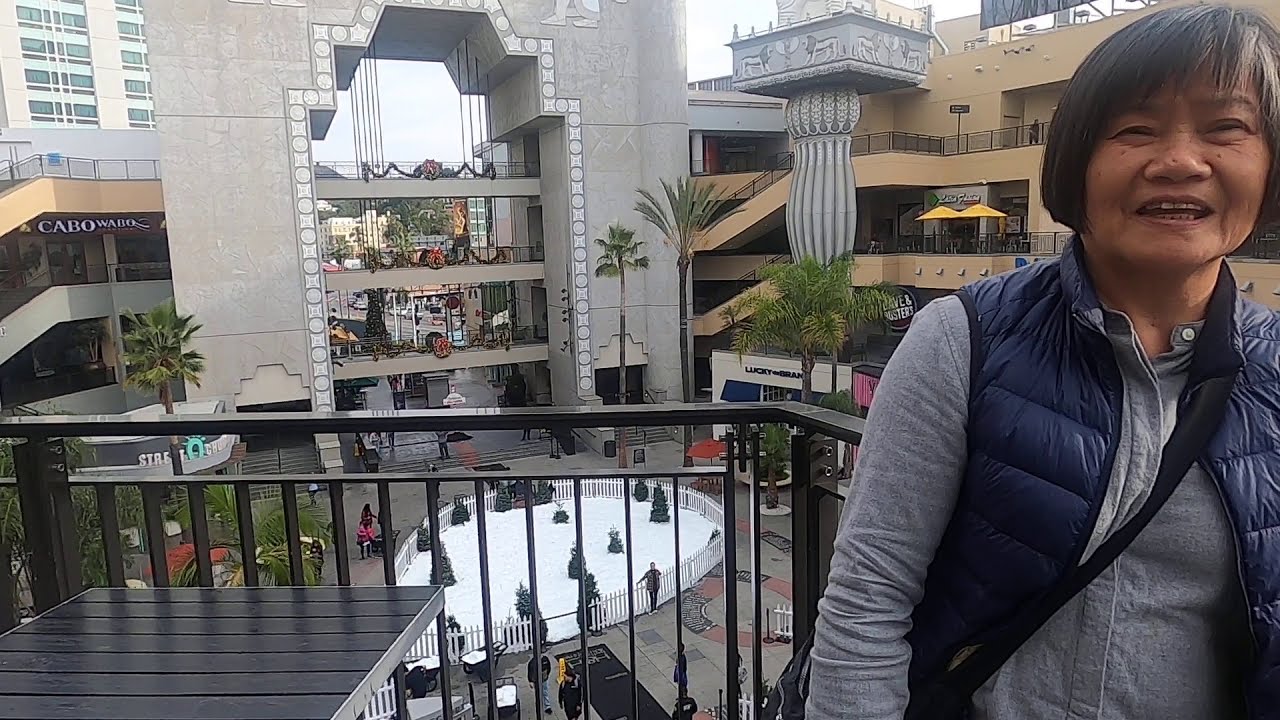The image depicts an elderly Asian woman, possibly Korean, standing on a balcony in a modern city square. She has short black hair with a hint of gray and is wearing a gray shirt underneath a blue insulated vest, suggesting a mildly chilly environment. A black strap from her purse is draped across her chest, with the purse resting by her right thigh. She is smiling warmly at the camera. The balcony, which features a black metal fence, is part of a multi-level complex with floors and viewing areas extending across a circular venue. Below, the city square or town square is bustling with people gathering around a notable white oval structure, possibly an ice skating rink or performance area. The surroundings primarily consist of brown and gray tones, complemented by modern architectural elements. The square is encapsulated by tall buildings and interconnected by a grand arch, giving it a cosmopolitan ambiance.